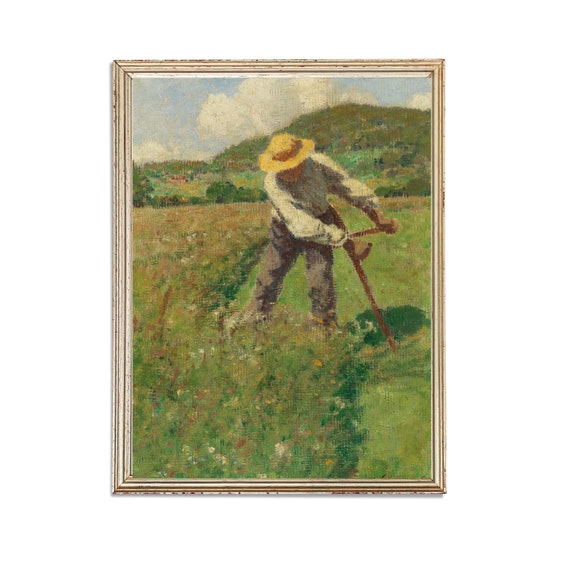This image features a small, intricately framed painting, capturing a moment of rural labor. The central figure is a man engrossed in the act of harvesting, poised in mid-swing with a long cutting tool. The contrast between the meticulously short-cropped grass behind him on the left (our right) and the tall, indistinct grass to his right (our left) emphasizes the progress of his labor. Clad in a long-sleeved white shirt, gray pants, and a brown straw hat that partially obscures his face, the man is depicted with a sense of focused determination. The background reveals lush, green hills under a softly clouded blue sky, enhancing the bucolic atmosphere and framing the scene with serene natural beauty.